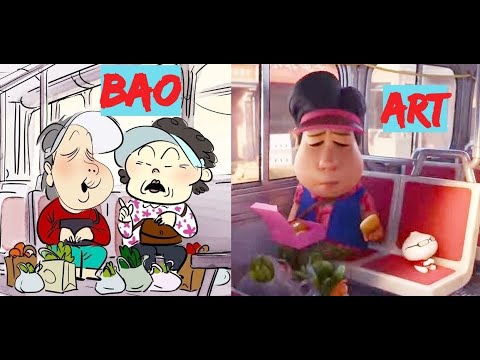This digital screenshot showcases two contrasting art styles side-by-side, both centered around public transportation scenes involving elderly individuals. The left half features hand-drawn art depicting an older couple sitting together amidst an array of grocery bags, with each wearing elaborate visors. The right half, rendered in a 3D art style, portrays an older woman seated alone, surrounded by groceries and a stuffed animal placed on the adjacent seat. The image prominently displays the text "Bau Art." The color palette primarily includes red and white, accented by pink, blue, and green hues. There are thematic parallels to the Disney short "Bao," which focuses on familial bonds, symbolized here by food items like a dumpling.